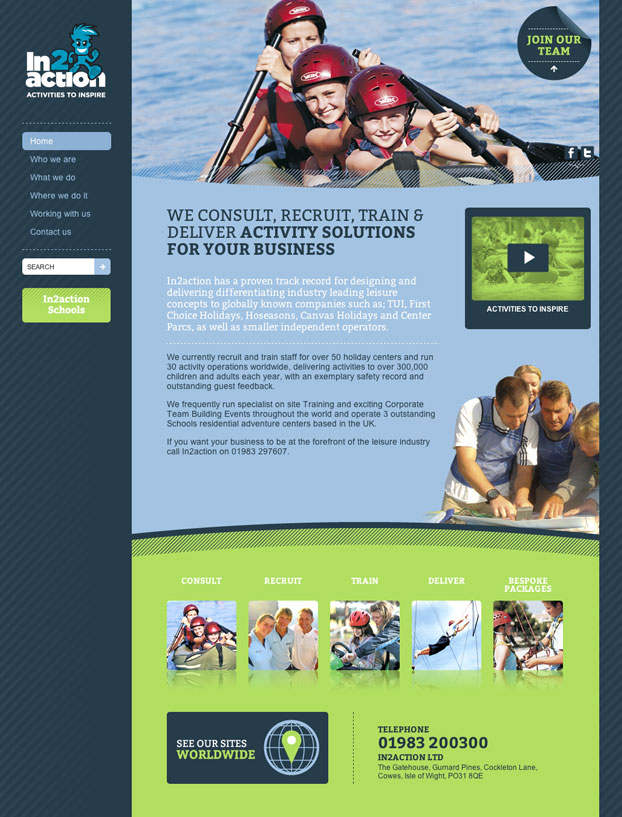The website presented serves as a hub for leisure activity solutions tailored for businesses. At the top of the page, the slogan "Actions to Inspire" is prominently displayed next to the company's logo. There is an engaging blue cartoon character with spiky hair that draws the viewer's attention.

The navigation bar includes various sections: "Home," "Who We Are," "What We Do," "Where We Do It," "Working With Us," "Contact Us," and a search bar. Just below, there's a section entitled "Into Action Schools" set against a green background with white text. A call to action invites users to join the team, with social media links for Facebook and Twitter nearby.

A featured image shows three people kayaking—two children and a woman—all wearing red helmets and using black paddles, emphasizing the company's active, outdoor focus. The caption underneath reads, "We consult, recruit, train, and deliver activity solutions for your business." 

"Into Action" highlights its track record of designing and delivering unique, industry-leading leisure concepts for globally recognized companies such as TUI, First Choice Holidays, O Seasons, Canvas Holidays, and Center Parcs, as well as for smaller independent operators. The company currently recruits and trains staff for 50 holiday centers, manages 30 activity operations worldwide, and serves over 300,000 children and adults annually, boasting a pristine safety record and outstanding guest feedback. Additionally, they offer specialist on-site training and corporate team-building events globally and operate three top-tier schools, residential, and adventure centers in the UK.

An additional section encourages businesses looking to lead in the leisure industry to contact "Into Action" at 01983 297. Next to this, an image shows two men and two women examining what looks like a map, capturing the consulting aspect of the business.

Below, sections labeled "Consult," "Recruit," "Train," "Deliver," and "Bespoke" showcase a variety of activities from boating to driving. There's also an interactive globe marked with green points, indicating the company's global reach. The footer includes the contact details: telephone 01983 200300, Into Action LTD, Gatehouse, Gurnard Pines, Cockleton Lane, Cowes, Isle of Wight, PO31 8QE.